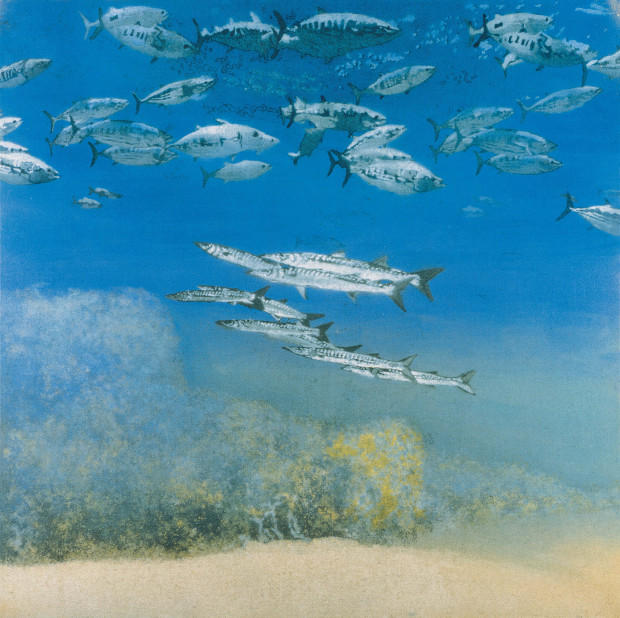The image shows an underwater scene with a vibrant and busy aquatic environment. At the top, a large, dense school of smaller, silverish-white fish swim collectively to the right, creating a sense of motion and unity. Contrasting this, a group of sleek, shark-like fish, possibly part of the broader school, are swimming in the opposite direction, lending a dynamic contrast to the image. Scattered throughout are varying sizes of fish, some slimmer and longer, all shimmering with hints of blue markings along their bodies. The ocean floor is plainly visible, covered in a layer of brownish sand, with spots of what appears to be yellow coral or plant life. Additionally, higher up in the scene amidst the fish, there is some taller vegetation, contributing to the image's depth and complexity. The background is a deep, calming blue, occasionally interrupted by whitish, cloudy formations that enhance the underwater ambiance.